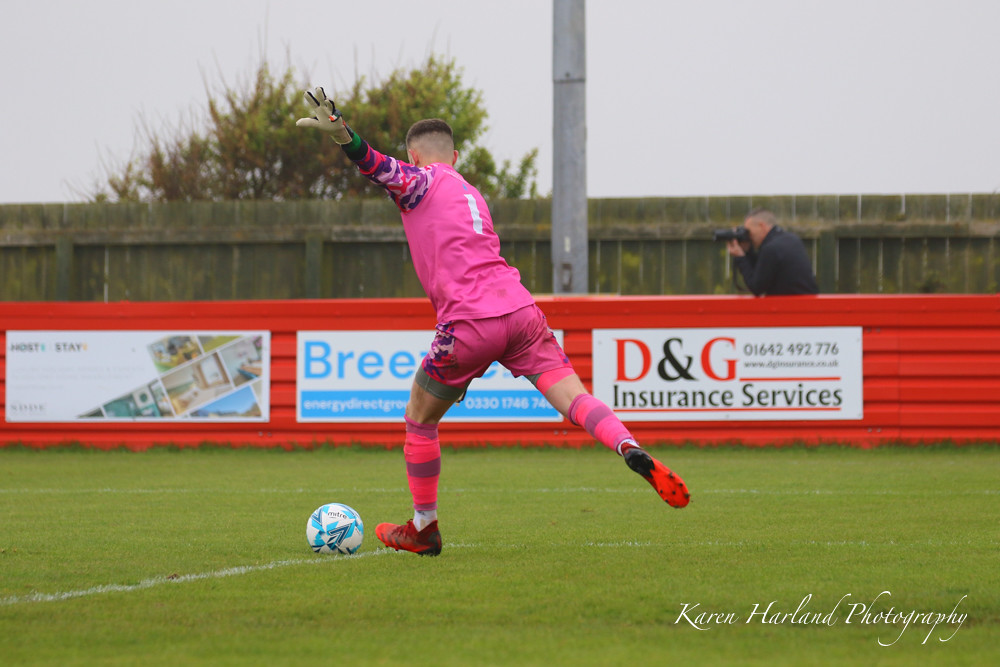This is a detailed photograph captured by Karen Harland Photography, showcasing a soccer player in mid-action just about to kick a white-and-blue soccer ball. The athlete is entirely focused, wearing a bright pink uniform with unique multicolored camouflage sleeves in shades of purple, pink, and red. His outfit includes matching pink shorts with a similar pattern on the leg, gray and pink leg protectors, pink and purple shin guards, and vibrant red shoes with cleats. The player also sports long white socks up to his knees and gloves, with his short hair clearly visible. The scene is set on a lush green soccer field, accented by a slightly blurred background featuring a wooden fence, tree, and several sponsor banners, including D&G Insurance Services and Breeze. Another photographer, with a camera in hand and wearing a dark sweater, can be spotted leaning against a red wall, focusing on another area. The bottom right corner of the photograph is marked with the logo "Karen Harland Photography."